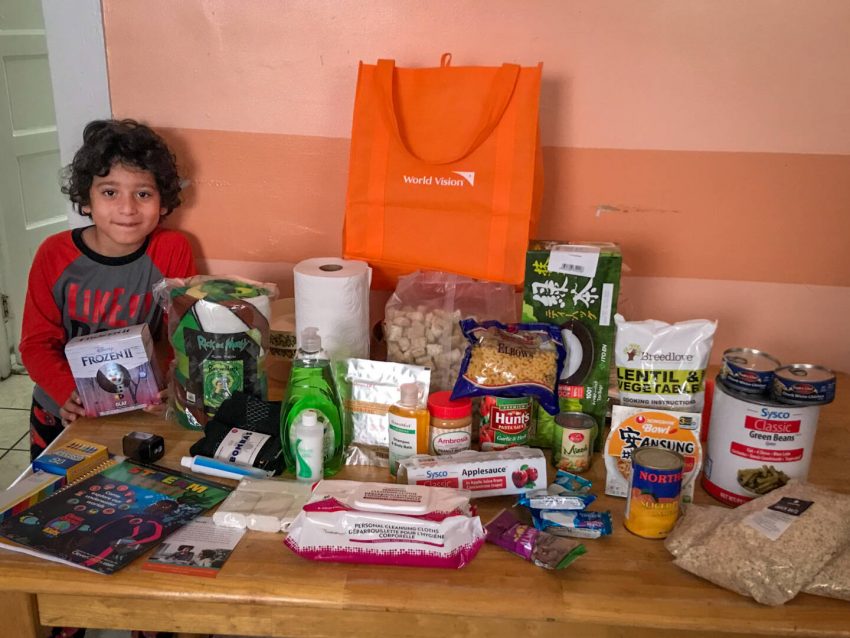A young boy with dark, curly hair and brown eyes stands smiling next to an oak wood table, loaded with a variety of groceries and household items. He is dressed in a gray shirt with red sleeves and the word "like" printed on it, alongside matching pajama bottoms. The background features a two-toned peach-colored wall with a horizontal stripe. 

On the table, there is a prominent orange tote bag labeled "World Vision." Surrounding the bag are numerous items, including canned goods like green beans, tuna, tomato sauce, and peaches, as well as dry foods such as elbow pasta and a bag of lentil and vegetable mix. Other groceries include a large bag of Frosted Mini-Wheats, individual servings of applesauce, a package of baby wipes, a roll of paper towels, dish soap, toothpaste, and hand sanitizer. 

The boy is holding a boxed toy from the Disney movie Frozen 2, featuring Olaf on the front. Additionally, there are personal care items such as a clear bottle of shampoo, a small container of ambrosia, and potential bags of either cereal or dried oatmeal. The presence of crayons and a coloring book adds a touch of whimsy to the scene, hinting at the child’s playful nature amidst the array of everyday necessities.